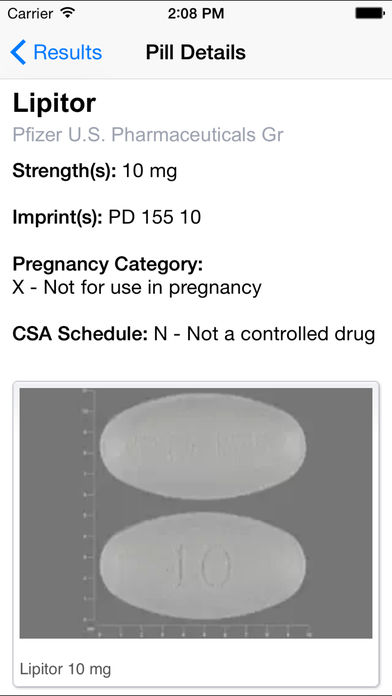The image features a detailed depiction of a Lipitor pharmaceutical product as follows:

- **Background**: The image is set against a white background.
- **Time Stamp**: The time displayed is 2:08 PM.
- **Color Scheme**: The results are highlighted in blue.
- **Drug Identification**: The pill shown is identified as Lipitor, manufactured by Pfizer U.S. Pharmaceuticals.
- **Imprint Details**: 
  - The pill has "Lipitor" imprinted on it in capital letters (L-I-P-I-T-O-R).
  - There is an imprint "S" in parenthesis, as well as "PD-155 10".
- **Dosage and Strength**: The pill is marked with "10 MG".
- **Pregnancy Category**: The drug is categorized under pregnancy category X, indicating it is not for use during pregnancy.
- **Controlled Substance Status**: 
  - The CSA (Controlled Substances Act) Schedule is listed as "N", signifying it is not a controlled drug.
- **Graphical Elements**: 
  - There is a chart included that likely relates to dosage or measurement, indexed from 0 to 10 on the bottom axis and from 0 to 11 on the left side.
  - The image features two pills; the first one is blank while the second pill has the number "10" engraved on it.

This caption provides a comprehensive and detailed description of the Lipitor drug product, its physical characteristics, regulatory information, and additional contextual details.